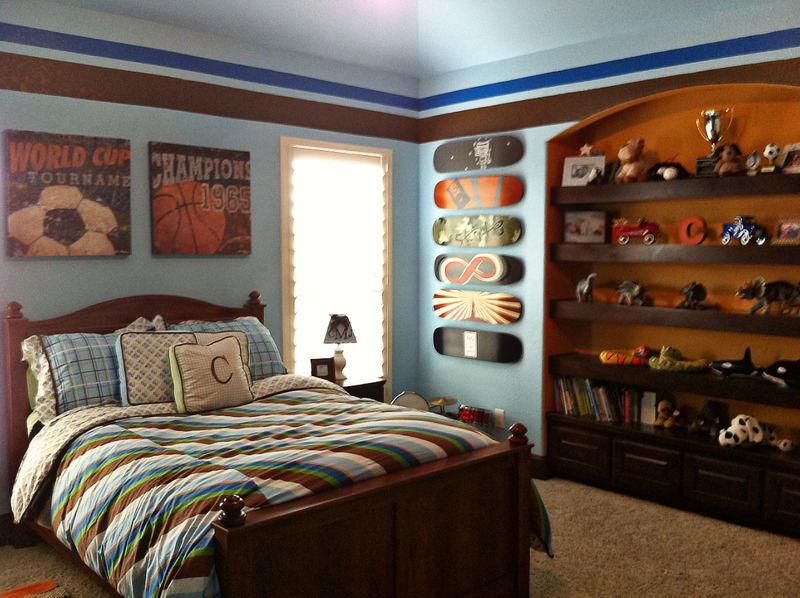This is a detailed photograph of a neatly organized, brightly lit bedroom, likely belonging to a boy. The room features a heavy mahogany wood bed with a headboard and footboard, adorned with a striped comforter in blue, green, and brown, complemented by two large pillows, three medium-sized pillows, one of which has the letter "C". The tan carpet adds warmth to the room, enhanced by sunlight streaming through a window. 

The walls are painted light blue with a brown border and a thin royal blue stripe running above it. Mounted above the bed are two posters, one depicting the World Cup Tournament and the other, Champions 1965, with a nod to soccer and basketball.

Prominently displayed on embedded wall shelves with an archway beneath, are an assortment of trophies, books, stuffed animals, model dinosaurs, and cars. To the right side wall, six skateboard decks in various colors—black, orange, green, striped red and white—are stacked vertically. An end table with a small lamp featuring the initials "CMJ" sits beside the bed. Overall, the room is a vibrant, personalized space characterized by its sky blue walls, sporty decor, and organized layout.